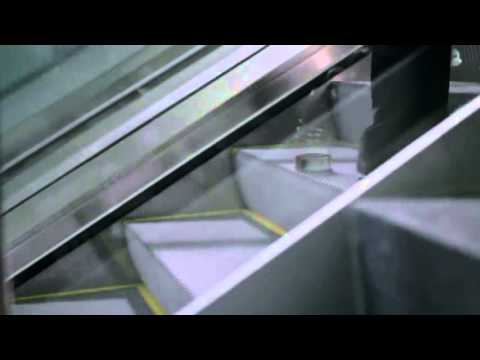This rectangular photograph showcases a silver escalator in a landscape view. The escaltor's steps are a light gray color with a subtle yellow border. In the top right corner, part of a person's leg in black pants is visible. The escalator, ascending diagonally from the bottom left to the upper right, is flanked by a light gray wall in the bottom right corner and another wall in the upper left corner. The image is framed by thick black bars at both the top and bottom, adding a cinematic touch to the composition.